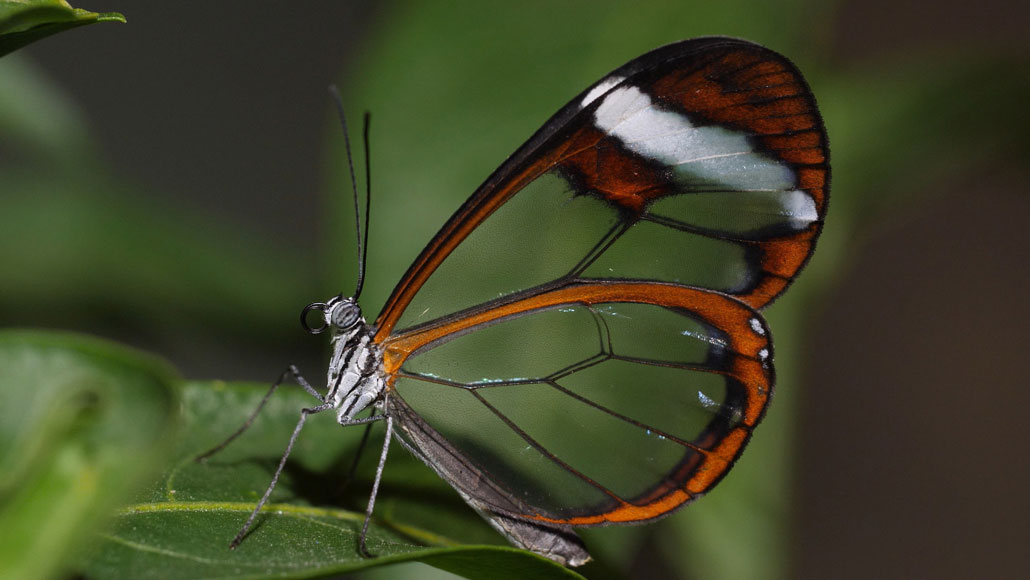This photograph features a unique and striking butterfly perched on a green leaf, set against a blurry background likely composed of more foliage. What sets this butterfly apart is its exceptionally clear wings. The majority of the wings are transparent, with only the edges and some intricate lines showing vibrant orange and black colors. The black and white striped body of the butterfly, reminiscent of a zebra pattern, adds to its distinct appearance. The butterfly is captured at eye level, staring directly at the camera, giving an intimate and detailed perspective. The clarity with which the delicate structures, like its antennae and the transparent parts of its wings, are rendered suggest this is a high-resolution, macro-scale shot. Although the exact time of day is uncertain, the sharpness and detail imply it could have been taken outdoors.